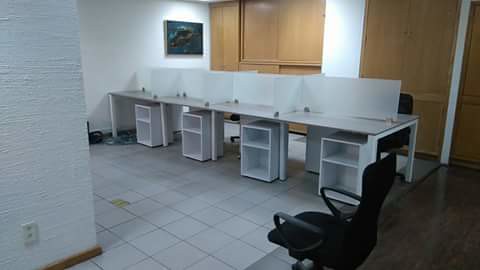The image showcases an empty makeshift office with a centrally located white desk divided into four cubicles. Each cubicle is designed to accommodate a computer but remains unoccupied. The desk features short white bookcases or small side tables beneath each division. The floor is primarily composed of white tiles, though a section of brown laminate wood flooring borders the tiles. The walls are white with brown baseboards, and against the back wall, there are light tan or brown wooden cabinets. A bluish-green picture is centered on the back wall, though its details are indistinguishable. Two black rolling chairs with armrests are positioned near the desk area, one at approximately the 5 o’clock position and the other on the opposite side. Additionally, a visible outlet is located on the right wall. The overall impression is of a sparse, utilitarian workspace waiting to be furnished.